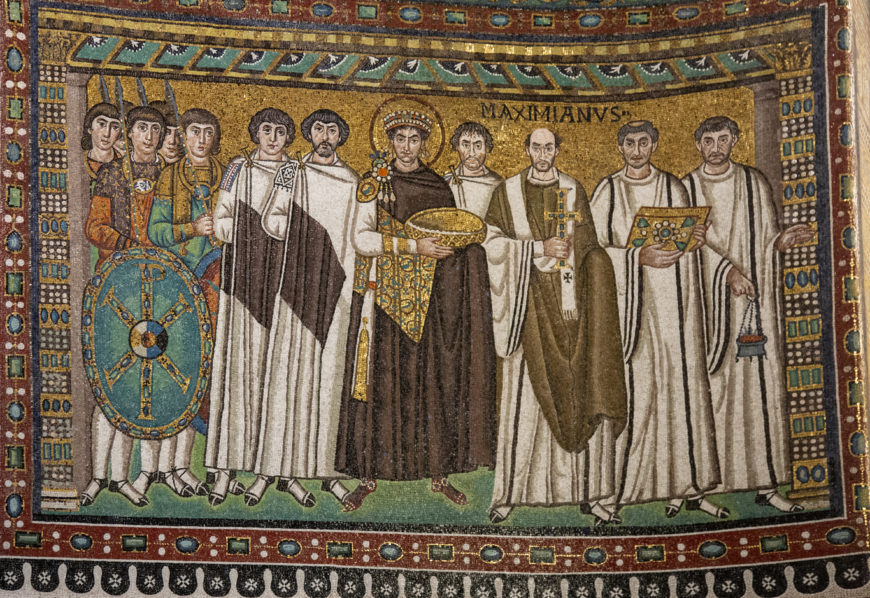The image appears to be an intricately detailed tapestry or mosaic dating back to Roman times, depicting a religious or ceremonial scene. At its center stands a prominent figure, possibly a king or priest, adorned in a dark brown and gold-embellished robe, holding a woven bowl. He is encircled by several men clad in floor-length beige, white, and brown robes, each holding various items such as a map, a cross embellished with green gems, a lantern, gold books, and a small bucket. The figures all share solemn expressions, and their detailed faces exhibit various hairstyles typical of the period. To the left, there are warriors holding shields, swords, and spears, with their garments appearing in shades of orange and green. The shield, notable for its teal and crisscross design with circular symbols, adds a bright contrast. The entire scene is framed by a lavish border in gold, greens, blues, and reds, with an inscription at the top reading "M-A-X-I-M-I-A-N-V-S".